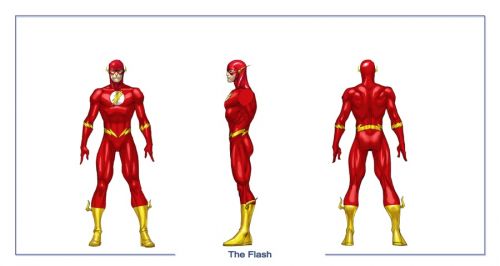The image is a detailed concept art of the superhero, The Flash. The rectangular artwork has a white background bordered by a thin light blue line. At the bottom center, the text "The Flash" is prominently displayed. The character is depicted in three different views: a front view on the left, a side profile in the middle facing left, and a rear view on the right. The Flash is clad in a skin-tight, candy-apple red outfit, complete with yellow boots that extend just below his knees, adorned with small lightning bolt designs. His outfit includes a red mask, and on his chest is a white circle emblem with a yellow lightning bolt. Additionally, there are lightning bolt bands around his forearms and one by his waist, emphasizing his signature speedster design in this striking and dynamic presentation.